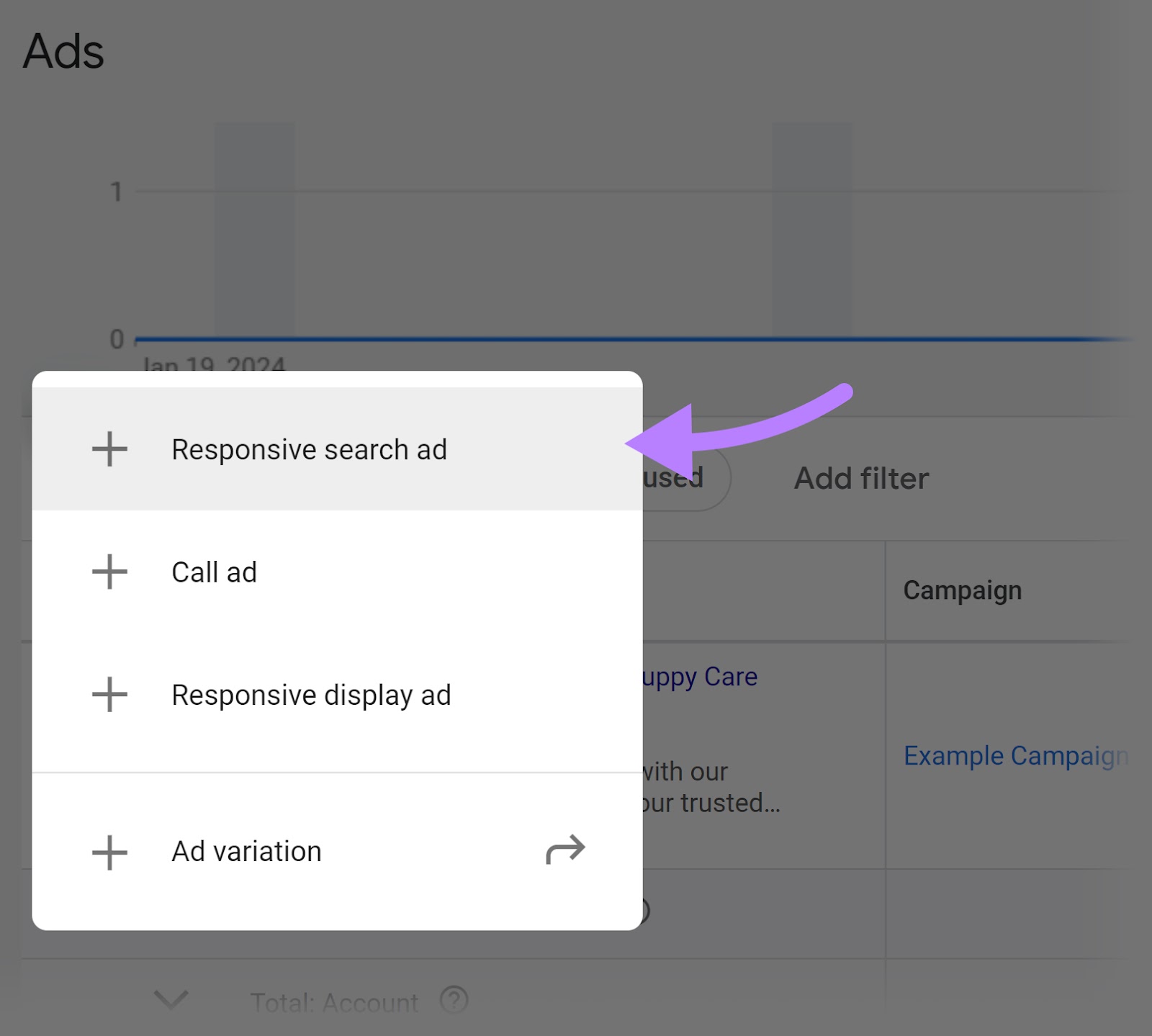In this image, we see a setup page for creating ads. The interface prominently displays four options for different types of ads: "Responsive Search Ad," "Call Ad," "Responsive Display Ad," and "Ad Variation." A purple arrow is clearly pointing towards the first option, "Responsive Search Ad," indicating it as the selected or recommended choice. Additional text labels include "Ad Filter," "Campaign," and an example campaign name, "Supply Care," which provide context for the setup process. The overall layout of the page is designed to guide users through selecting and configuring their ad preferences efficiently.